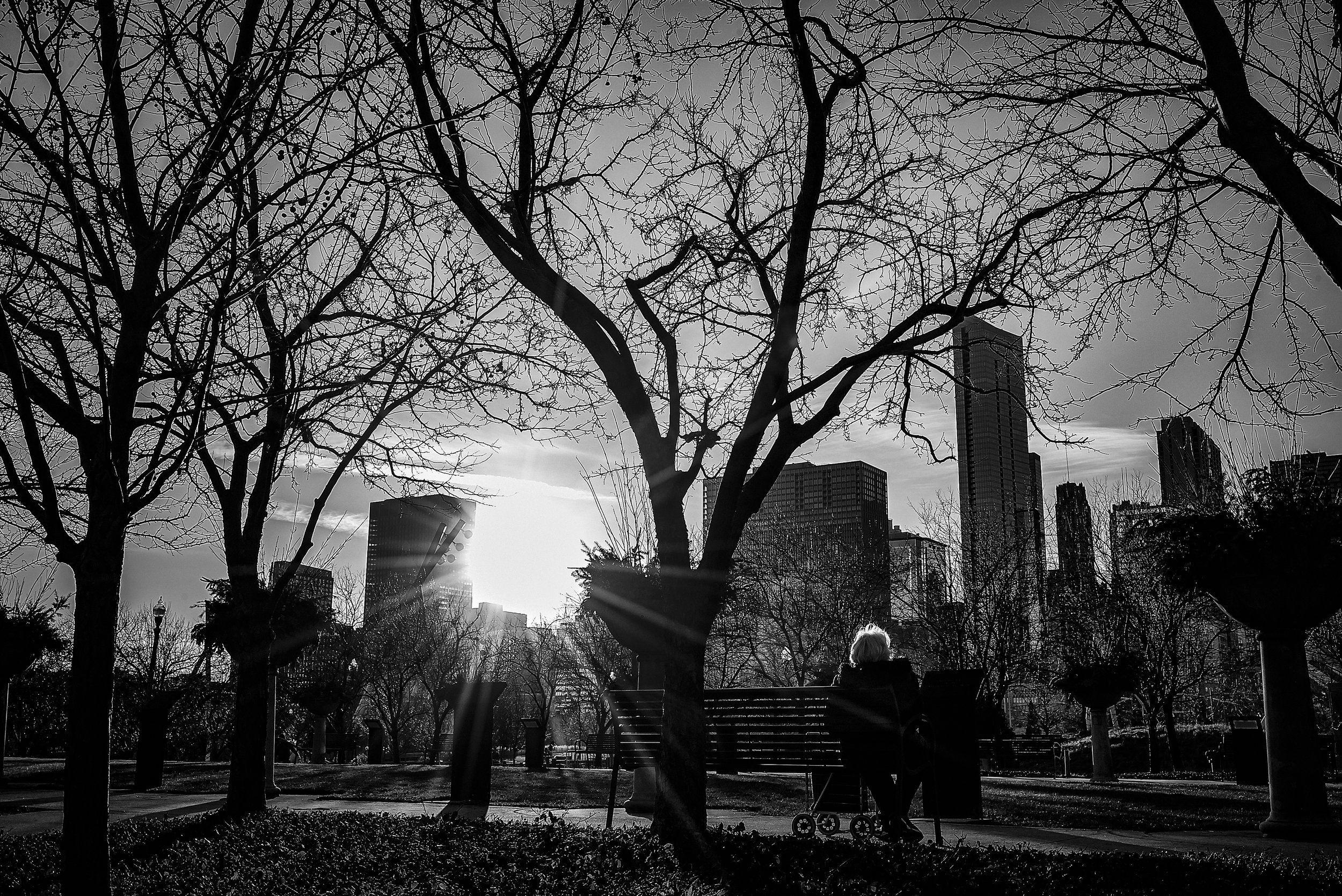This captivating black and white photograph captures a serene moment in an urban park on a clear, sunny yet wintry day. In the foreground, we see a grassy area just behind a lone park bench, where an elderly woman with short, white hair is seated, gazing toward the distant cityscape. To her left, a small wagon cart is nestled next to the bench. The park is dotted with several tall trees devoid of leaves, hinting at the late autumn or winter season. The skyline behind the park features an array of towering skyscrapers and rectangular buildings, with the sun brilliantly shining through, creating high-contrast highlights and casting radiant sun rays across the scene. Sparse, wispy clouds embellish the bright sky, adding to the tranquil yet poignant atmosphere of the image.